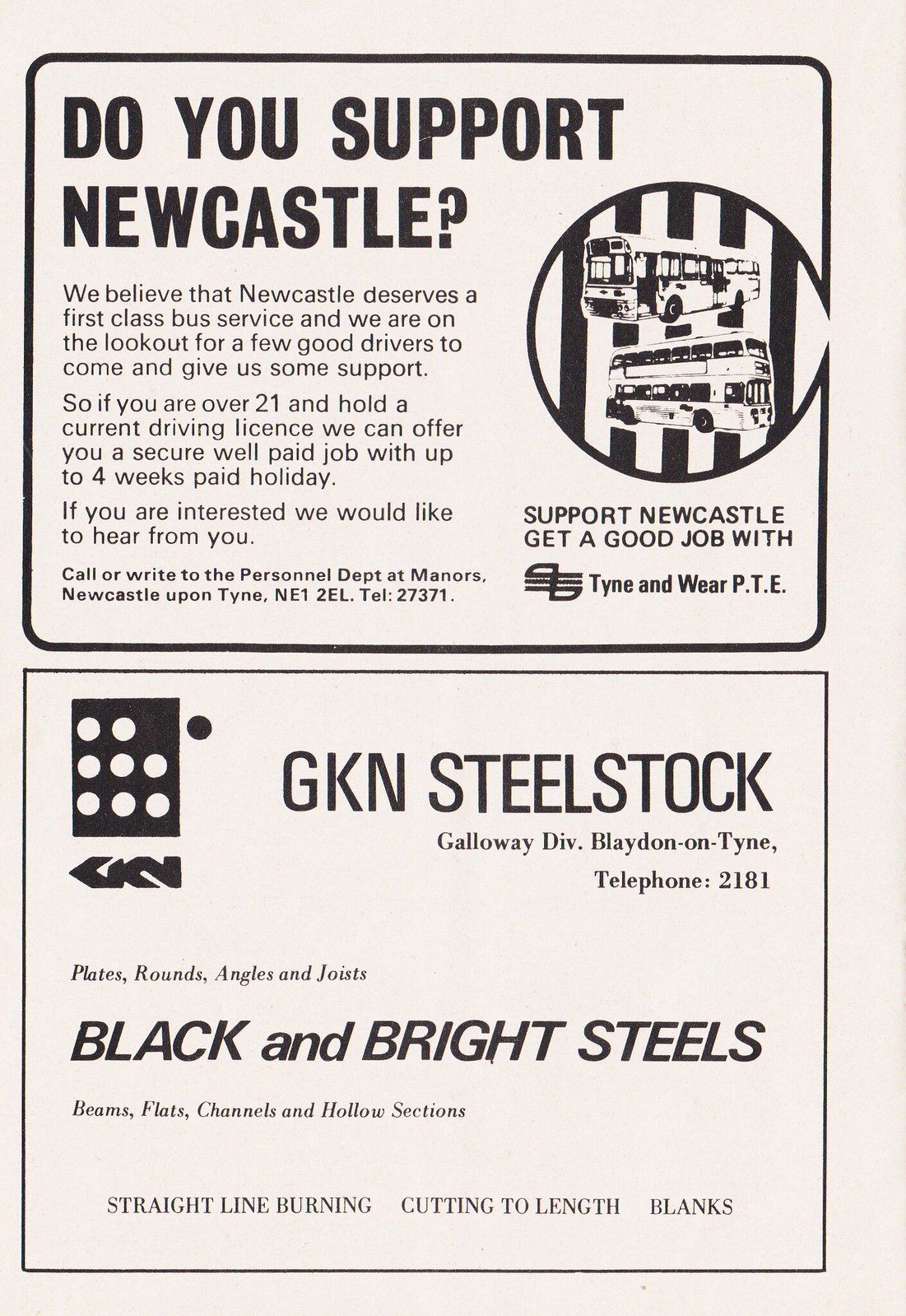The image is a compelling vintage advertisement on beige paper, divided into two distinct sections, each bordered by black rectangular frames. The top ad features a prominent headline in bold text, "Do you support Newcastle?" Accompanying this is a cartoonish depiction of both single-decker and double-decker buses with black stripes on a circle located on the right side. The ad advocates for Newcastle's first-class bus service and actively seeks drivers, offering a secure, well-paid job with up to four weeks of paid holiday for applicants over 21 with a current driving license. Interested individuals are encouraged to contact the personnel department at Manners, Newcastle upon Tyne, NE1-2EL, or call 27371. Below this, another ad promotes GKN Steel Stock, specifying their Galloway Division in Bladen-on-Tyne. It lists their telephone number as 2181 and details their offerings, including plates, rounds, angles, joints, black and bright steels, beams, flats, channels, and hollow sections. The company also provides services like straight-line burning and cutting to length.